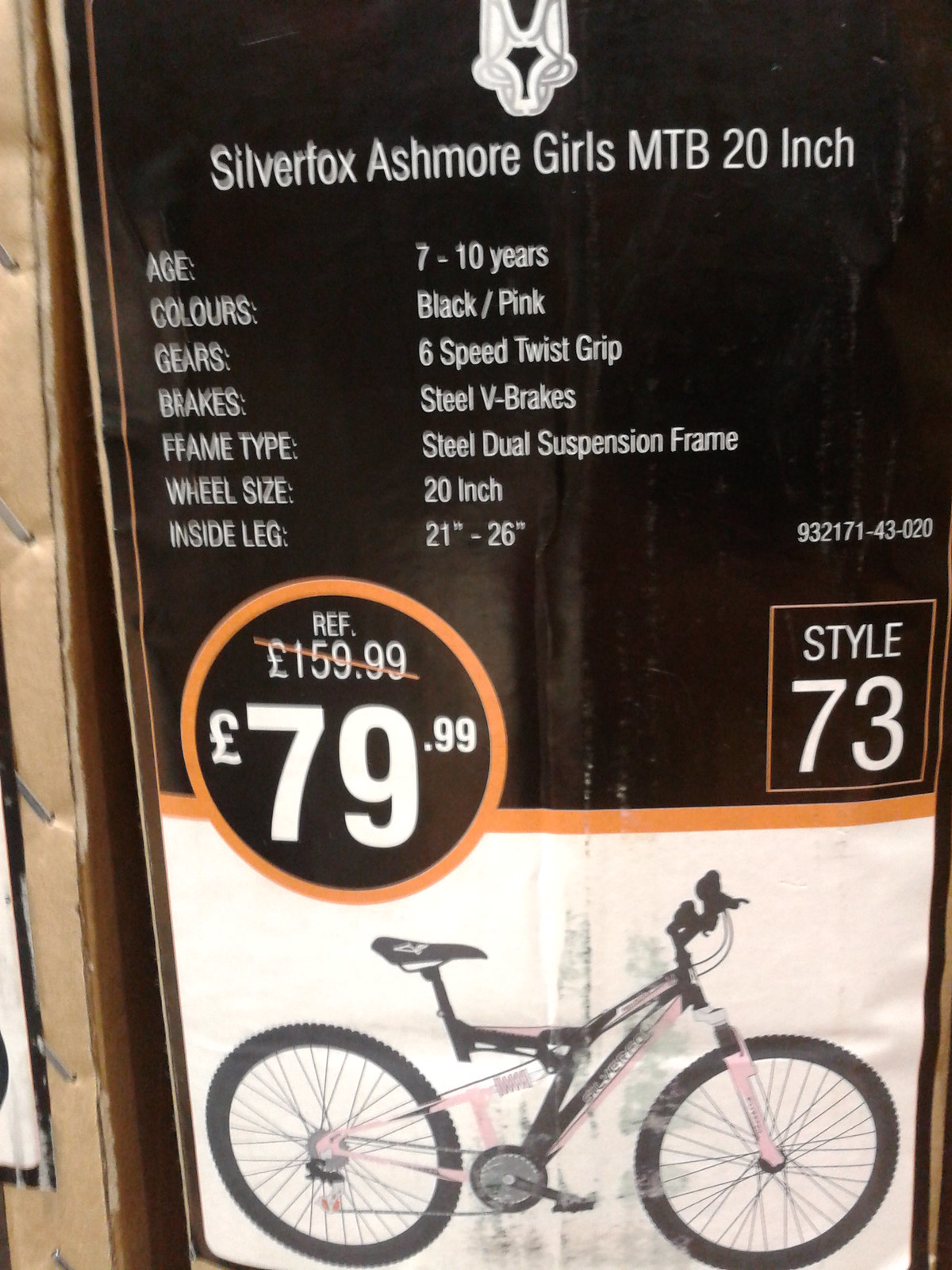This rectangular label is taller than it is wide and is affixed to a cardboard box. The top half of the label features a black background with white print. At the top center is the outline of a fox’s head, beneath which it reads "Silver Fox Ashmore Girls MTB 20-inch." Directly below this, the bike's specifications are listed in two columns: left and center. They include: "Age: 7-10 years," "Colors: black/pink," "Gears: 6-speed twist grip," "Brakes: steel V-brakes," "Frame Type: steel dual suspension frame," "Wheel Size: 20-inch," and "Inside Leg: 21-26 inches." Additionally, the far right of this section displays the numbers "932171-43-020."

Below, a horizontal orange line separates the top black half from the bottom white half. The bottom white section features an image of the mountain bike, showcasing its black and pink color scheme with visible seat, handlebars, wheels, and pedals. Above the image, on the left, is a black circle outlined in orange with "REF" inside, showing the original price of "159.99 pounds" crossed out in orange, and directly below, the sale price of "79.99 pounds" in large white numbers. To the right, in an orange-bordered black box with white print, it states "Style 73."